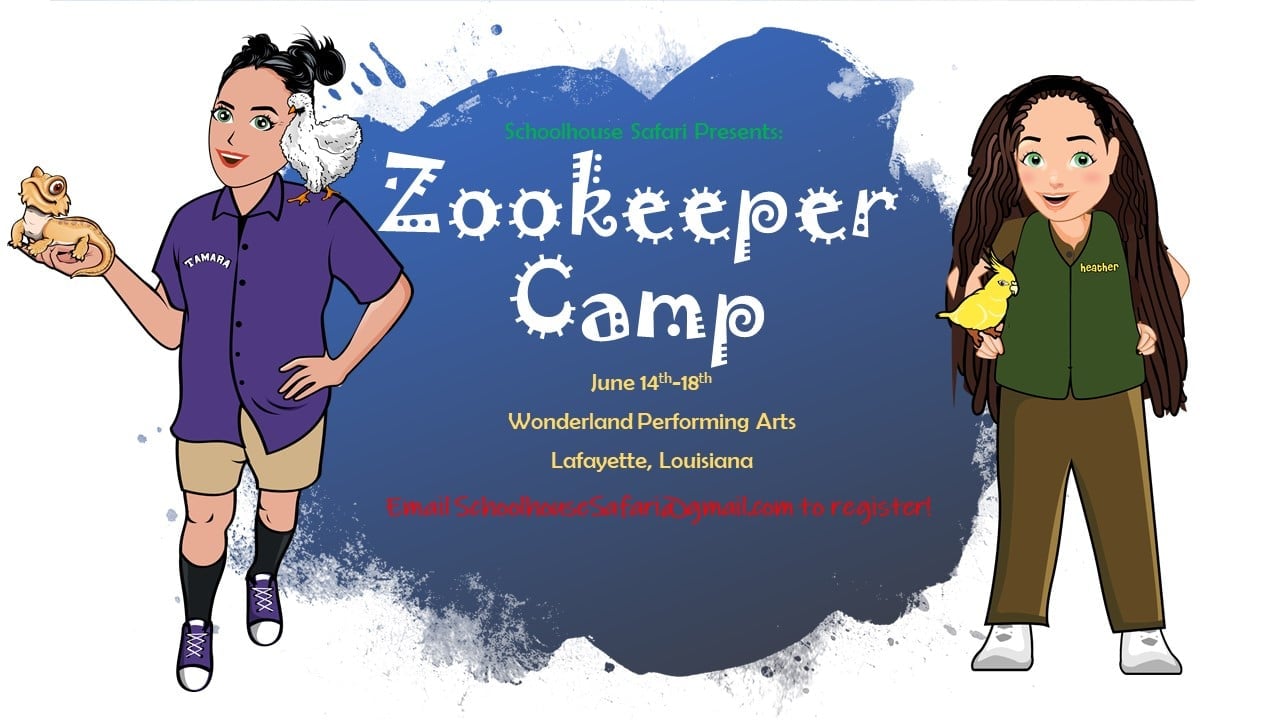The image is a colorful cartoon graphic design promoting the "Zookeeper Camp" organized by Wonderland Performing Arts in Lafayette, Louisiana, from June 14th to 18th. The image features two female characters standing side by side, facing the viewer. On the left is Tamara, identified by her name on her purple shirt. She has dark hair, green eyes, and a cheerful smile. Tamara is dressed in beige shorts, black socks, and purple high-top sneakers. Notably, she has a chicken perched on her left shoulder and is holding a lizard in her right hand. On the right stands Heather, who has long, wavy dark brown hair and green eyes. She is wearing a forest green vest with her name on it, paired with dark brown khaki pants and white sneakers. Heather is posed with her left hand on her hip while holding a cockatiel in her right hand. In between the characters, the text announces the details of the camp, along with an email address for registration, set against a blue background. The art style resembles Bitmojis, enhancing the whimsical and engaging feel of the advertisement.